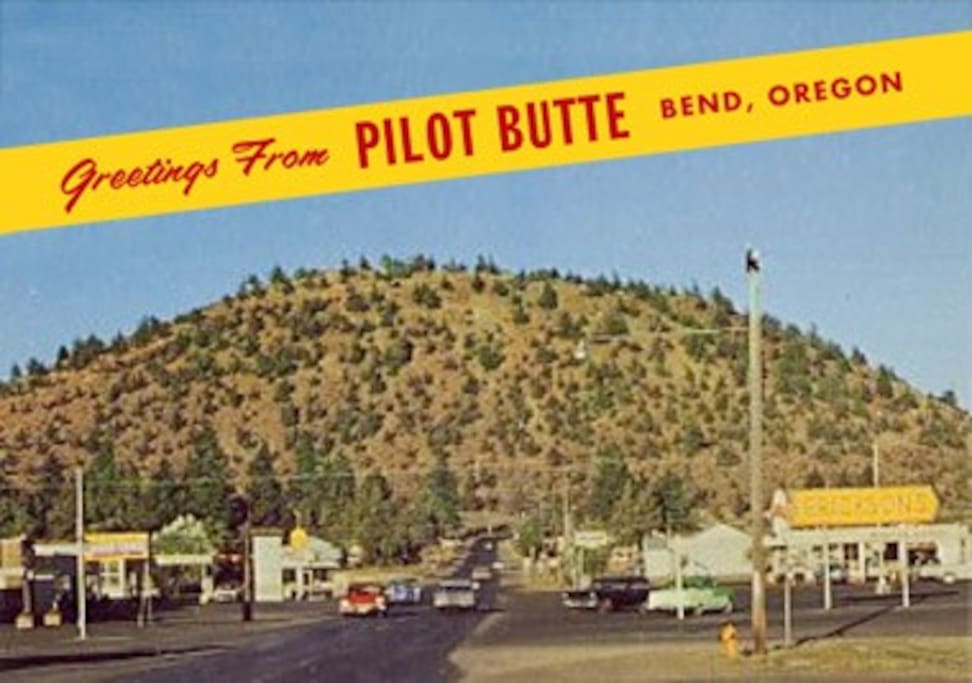This image appears to be an old postcard featuring a picturesque outdoor scene with an emphasis on nostalgia. A yellow banner with red cursive text reading "Greetings from Pilot Butte, Bend, Oregon" spans the top of the image. The background showcases a vast, brown circular hill dotted with numerous small pine trees, leading up to a clear blue sky. Below the hill, a quaint and old-fashioned town unfolds. The town is characterized by a single road lined with vintage 1950s-style cars and several indistinct small businesses, including what looks like a gas station and possibly a motel with a parking lot where two cars are parked. The overall atmosphere is imbued with an antiquated charm, highlighted by the faded colors and blurred details, indicative of a bygone era. The primary colors in the image include black, white, brown, green, red, yellow, blue, and gray, further enhancing its vintage postcard appeal.